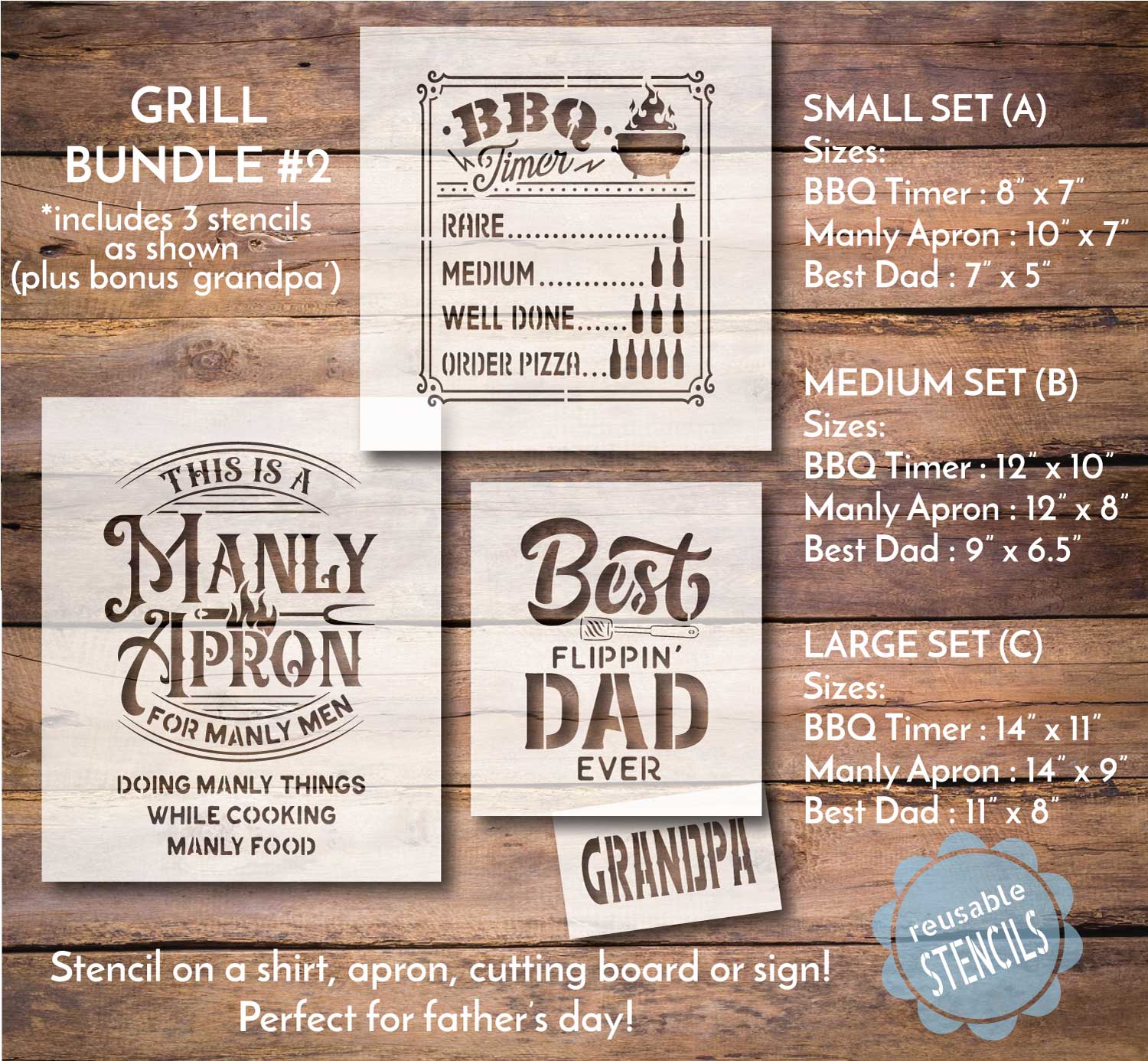This advertisement for reusable stencils features a detailed display on a rustic wooden plank background. The central element, "Grill Bundle Number Two," includes three stencils plus a bonus grandpa stencil. Highlighted stencils are "BBQ Timer" - illustrating cooking stages from rare to order pizza alongside corresponding beer bottles, "Best Flippin' Dad Ever" - which includes a spatula, and "Manly Apron" - proclaiming manly traits associated with grilling. Detailed measurements for each stencil are meticulously listed on the right, across three size sets: small, medium, and large. The small set includes a BBQ timer (8x7 inches), manly apron (10x7 inches), and best dad (7x5 inches). The medium set includes a BBQ timer (12x10 inches), manly apron (12x8 inches), and best dad (9x6.5 inches). Finally, the large set includes a BBQ timer (14x11 inches), manly apron (14x9 inches), and best dad (11x8 inches). A blue seal confirming the stencils' reusability adorns the bottom right, enhanced with petal-like accents. Another clear label on the bottom of the display recommends using these stencils on shirts, aprons, cutting boards, or signs, making them perfect Father's Day gifts.